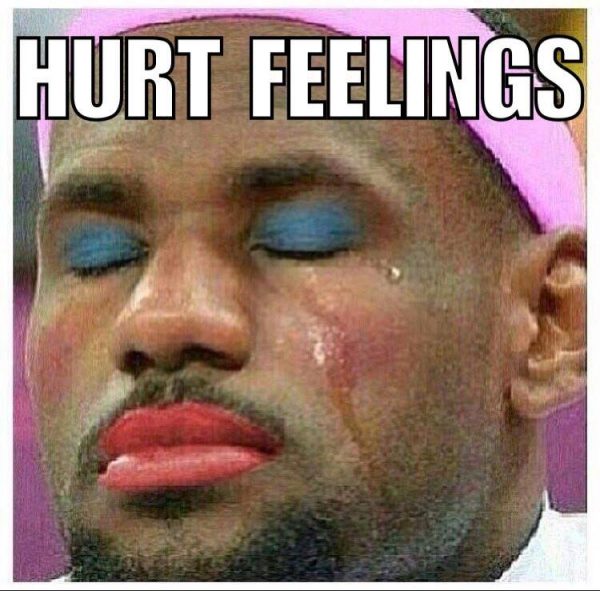The image is a close-up of a digitally altered photograph of LeBron James, set against a pink background. LeBron’s eyes are closed, with clear tears streaming down his left cheek, indicating that he is crying. His makeup includes bold blue eyeshadow on his eyelids and bright red lipstick. He has notable facial hair, including a goatee, and wears a bright hot pink headband. The image captures the upper portion of his white shirt. Across the top of the image, in bold white capital letters with a black outline, the text "HURT FEELINGS" is prominently displayed, reflecting the meme's theme.